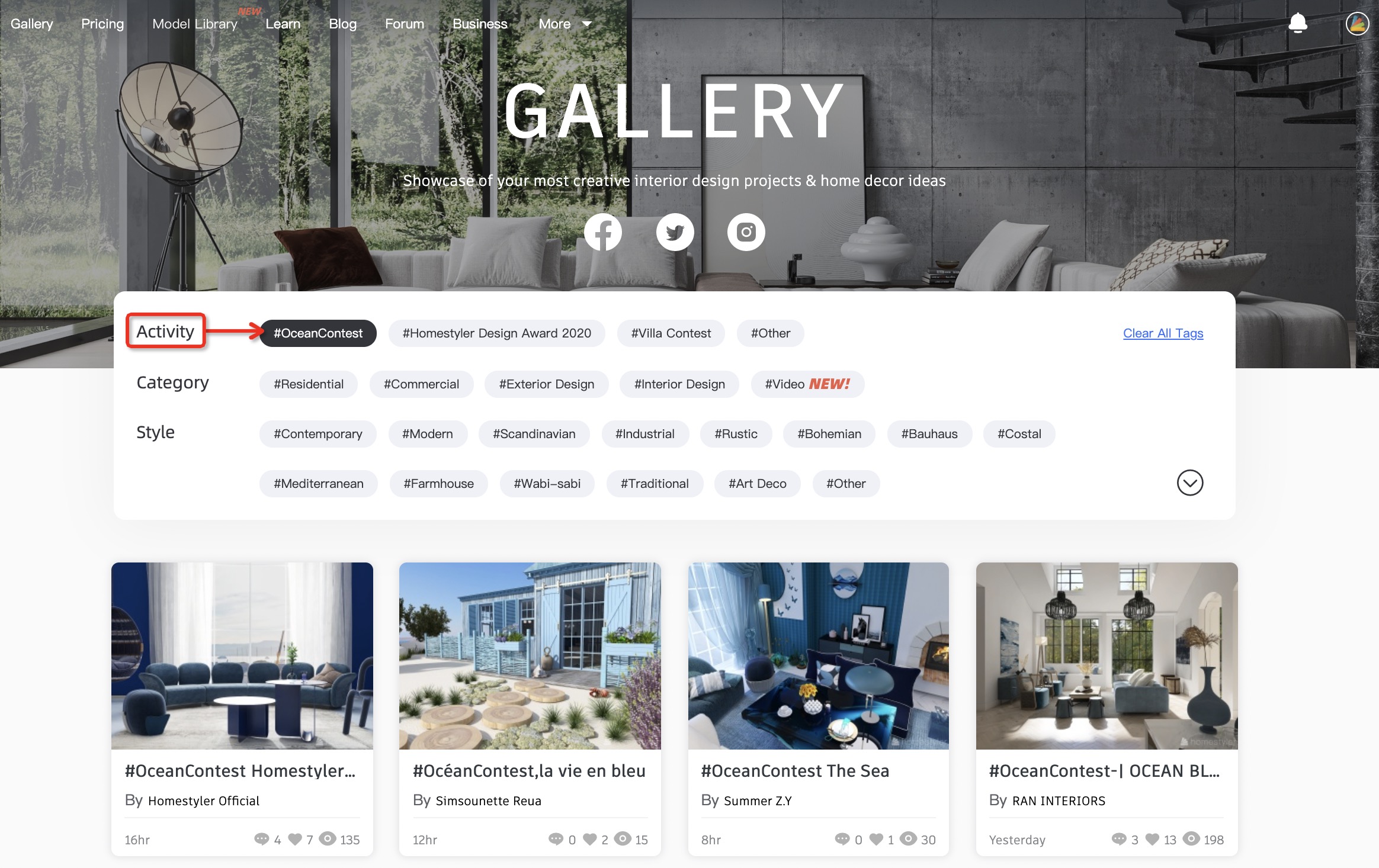**Caption for Image:**

This is a detailed screenshot of an e-commerce web page focused on interior design. The top third of the page is dominated by an image showcasing a modern, stylish interior living space. In the center of this image, the word "Gallery" is prominently displayed in large, bright white text. Below this title, a subtitle reads, "Showcase of your most creative interior design projects and home decor ideas."

In the top left-hand corner of the page, a navigation menu lists various sections: Gallery, Pricing, Model Library, Learn, Blog, Forum, Business, and an option for more categories. Directly under the "Gallery" label, there are icons for Facebook, Twitter, and Instagram, indicating options for social media integration.

Further down, a section labeled "Activity" is highlighted with a red circle and arrow, suggesting its importance. Beneath this, a list appears with "Ocean Contest" in bold black, followed by "Home Style Design Award," "Via Contest," and "Other."

A categorized menu follows, featuring options such as Residential, Commercial, Exterior Design, Interior Design, and a new category named Video. Another filter allows users to select from various styles, including Contemporary, Modern, Scandinavian, Industrial, Rustic, Bohemian, Bauhaus, Coastal, Mediterranean, Farmhouse, Wabi-Sabi, Traditional, Art Deco, among others.

Below these detailed options, the page presents four images showcasing different types of homes and furnishings, each representing diverse interior design styles.